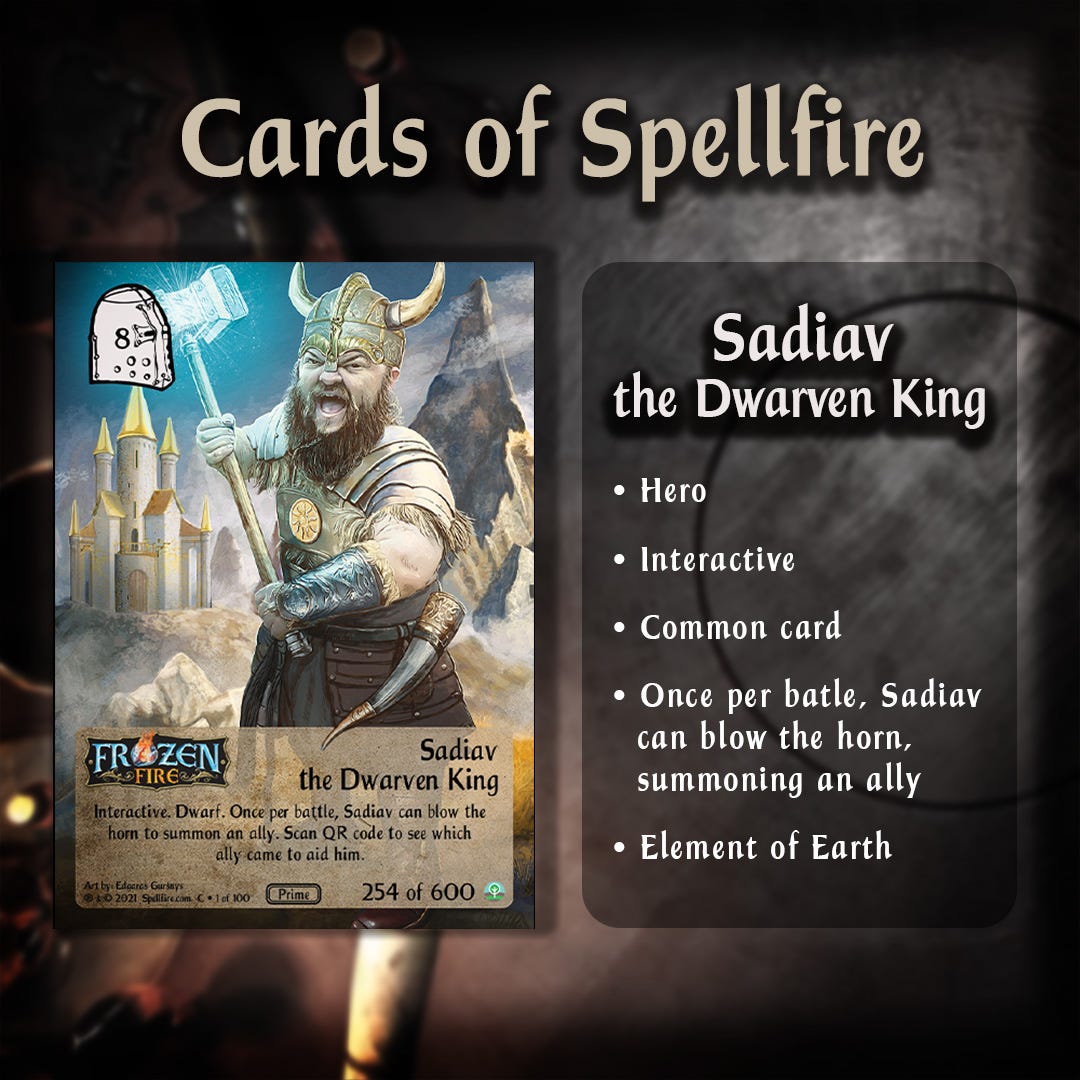This digital illustration serves as an advertisement for the "Cards of Spellfire" game. Set against a brown background, the top of the image prominently features the game's title in light brown letters. On the left side, there's an intricate illustration of Sadiab, the Dwarven King, a fantasy dwarf with a horned helmet, a long brown beard, and a viking-style outfit. He wields a sparkly axe and is depicted with a sneer on his face. Behind him stretches a majestic castle with golden roofs, set against a mountainous background. Below the character, the text identifies him as "Sadiab, the Dwarven King" and includes a tagline, "Frozen Fire." The card is interactive, allowing Sadiab to blow a horn once per battle to summon an ally, the details of which can be accessed by scanning a QR code. The term "Prime" appears beneath this ability description. At the bottom left, the card is labeled as "254 of 600," accompanied by a green icon. To the right of the character illustration, a text box provides additional information, describing Sadiab as a hero, interactive, a common card, and aligned with the element of Earth. The detailed formatting and specific attributions make it evident that this image is a part of a collectible card game, "Cards of Spellfire."